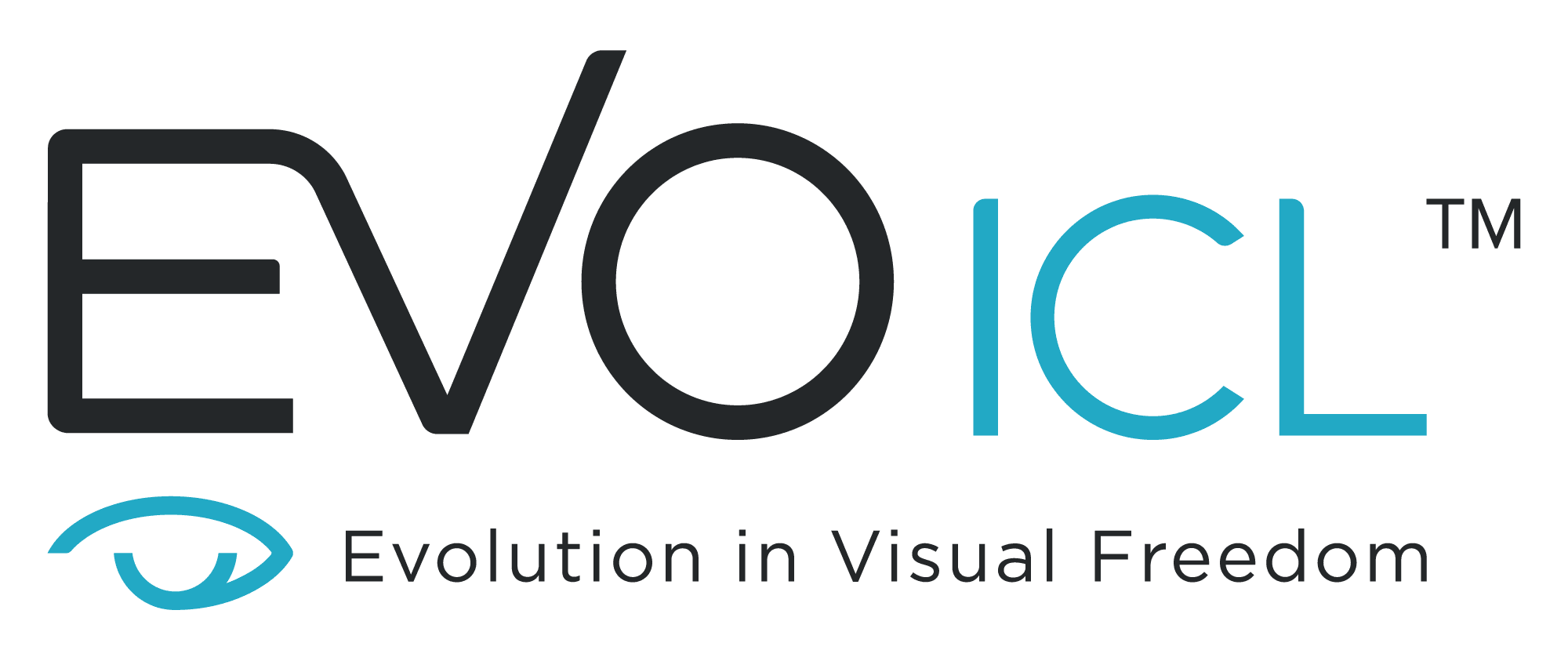The image is a company logo on a white background. Prominently displayed in large black capital letters is "EVO," followed by "ICO" in a bluish-green or teal color. In the upper right corner, a trademark symbol ("TM") appears in black. Below this text, there is an outline of an eye, also in the same teal color, shaped almost like an oval but curving in slightly on the left. Underneath the eye symbol, in black non-capitalized letters, it reads "evolution in visual freedom." The overall design suggests it is an advertisement for a brand related to eye care, possibly offering products or services such as contact lenses, eye surgery, or other visual freedom solutions. The seamless combination of the letters in "EVO" and the distinct separation of "ICO" with the eye symbol support the branding identity.